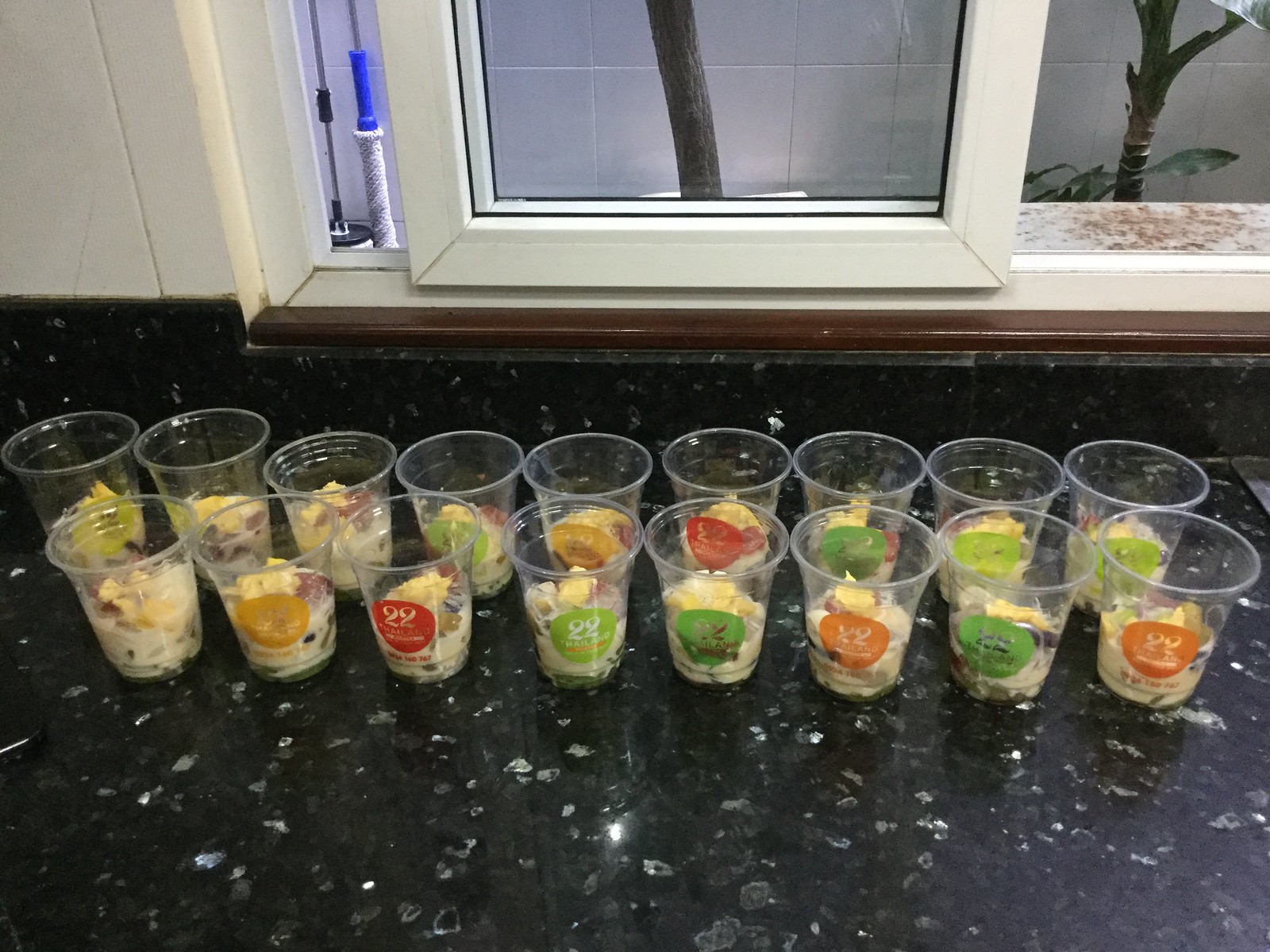The image depicts a black granite countertop with white and gray specks, set against a white wooden wall. To the right, there is an open two-pane sliding window with a white frame, revealing an outside view with slender tree trunks and some potted plants on a tiled surface. On the countertop, organized in two horizontal rows, are around 17 to 20 clear plastic disposable cups, each adorned with a circle design in red, green, or orange with the number "22." The cups contain small servings that appear to be an assortment of colorful appetizers, vegetables, or fruit and dip, including a red tomato-like disc, something white, something yellow, and a small slice of green kiwi. The scene hints at someone preparing for a gathering, possibly in a home or restaurant setting.